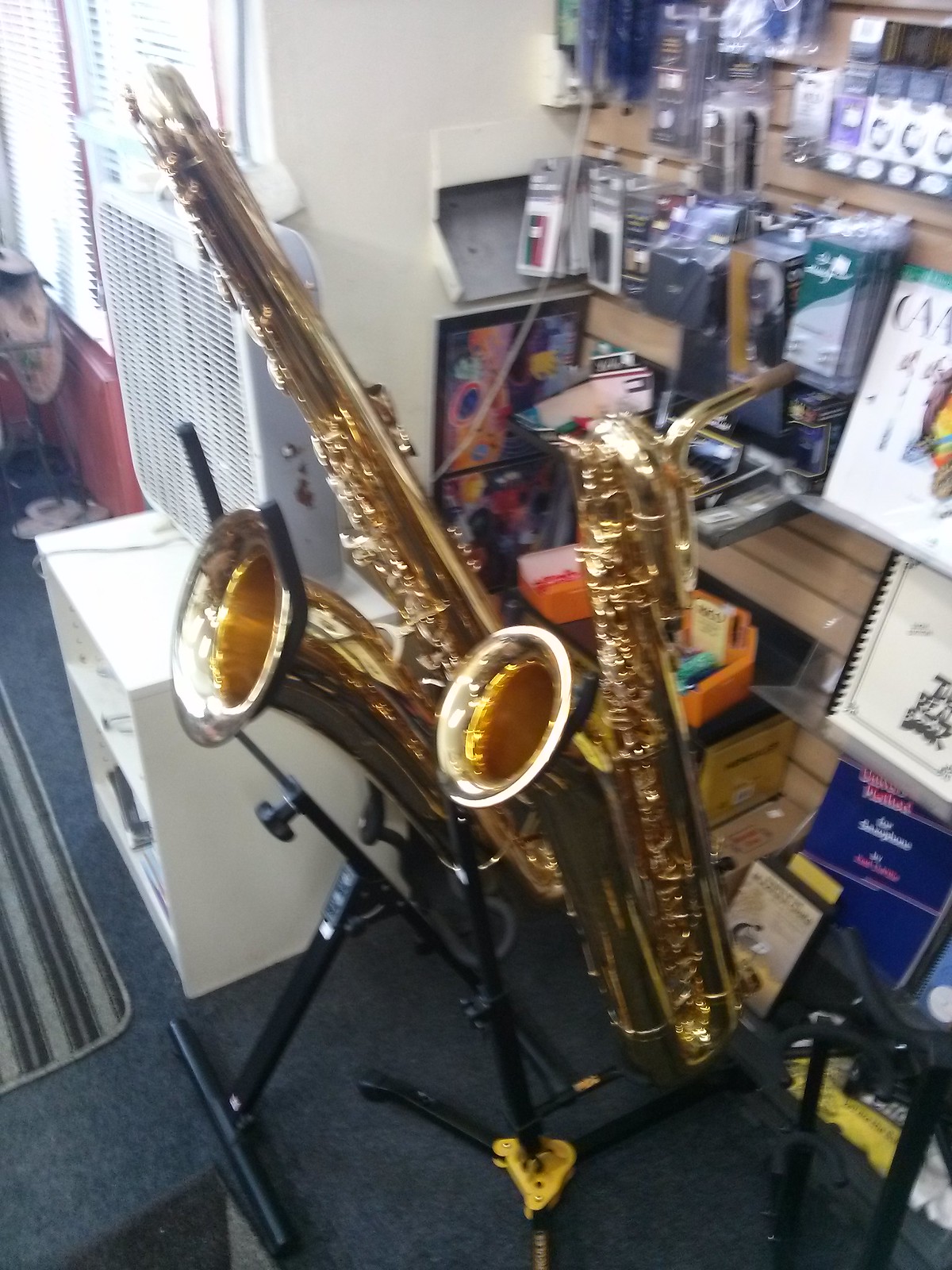This color photograph captures the interior of a musical instrument store, with a focus on two prominently displayed saxophones. The saxophones, one long and one short, are both gold and set on sturdy black stands with rubber-cushioned metal supports, ensuring the instruments are safely held at the tube portion. The longer saxophone features a less pronounced curve compared to its shorter counterpart. Both saxophones boast intricate embroidery and shine brightly under the store's lighting.

In the backdrop, there are wooden slapboard shelves holding various items mounted on pegs, though these are slightly out of focus, adding depth to the scene without distracting from the central subjects. To the right of the saxophones, a kiosk displays a variety of strings, brochures, and how-to books.

The store's ambiance includes a dark blue carpet, accentuated by a light gray rug with black and dark gray stripes, positioned in front of a small white stand. This stand, equipped with two shelves, supports a white box fan. The overall image, while slightly blurry and not of optimal quality, effectively conveys the rich, detailed environment of a well-stocked musical instrument store.